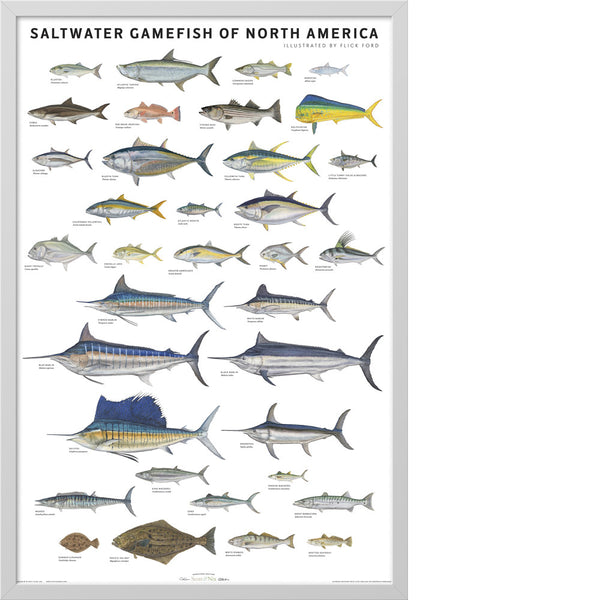The poster, titled "Saltwater Game Fish of North America," features a collection of approximately 20 to 30 vividly colored, almost cartoon-like drawings of various saltwater game fish. Displayed against a solid white background with a light gray border, each fish is shown in a side profile, facing left with their tails toward the right side. The centrally located swordfish, with their distinctive long, sword-like noses, stand out among the illustrations. The fish vary significantly in size, shape, and color, ranging from silver, blue, and brown to yellow. Noteworthy details include a blue fish with a feathery-looking fin on the lower left side and other fish with spiky blue fins along their backs. At the top of the poster, the title "Saltwater Game Fish of North America" is written in bold black capital letters, with "Illustrated by Flick Ford" in smaller print to the right. The largest fish are predominantly in the center and towards the bottom, while the smallest are often found in the corners, particularly the lower right.